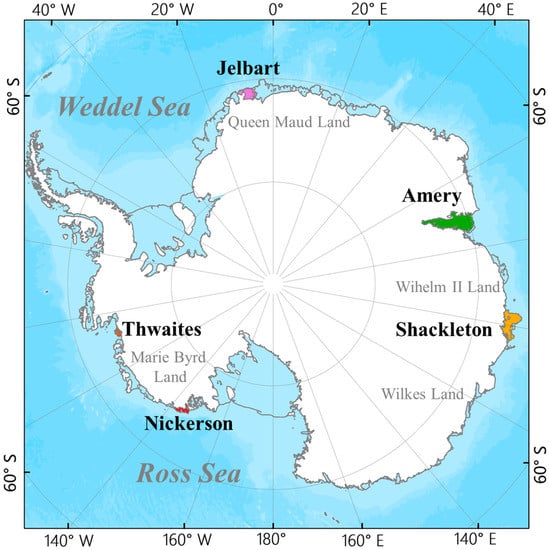This image is a detailed map of Antarctica, with the Weddell Sea labeled in the upper left and the Ross Sea in the bottom left. The landmass is primarily depicted in white, surrounded by blue to represent water. The map is bordered by coordinates: 40 degrees west to 40 degrees east along the top, and 20 degrees increments along the sides. Various regions are highlighted in distinct colors: Shackleton in orange, Amery in green, and Gelbart in pink at the top. Nickerson, highlighted in red, is at the bottom left. Additional named areas include Wilkes Land, Marie Byrd Land, and Queen Maud Land. Major landmarks such as Thwaites in brown and William II Land are also marked. The map emphasizes the central part of Antarctica, highlighting its coastline and surrounding islands. Directions are clearly indicated around the frame of the map, providing a comprehensive overview of the continent's geographical features.